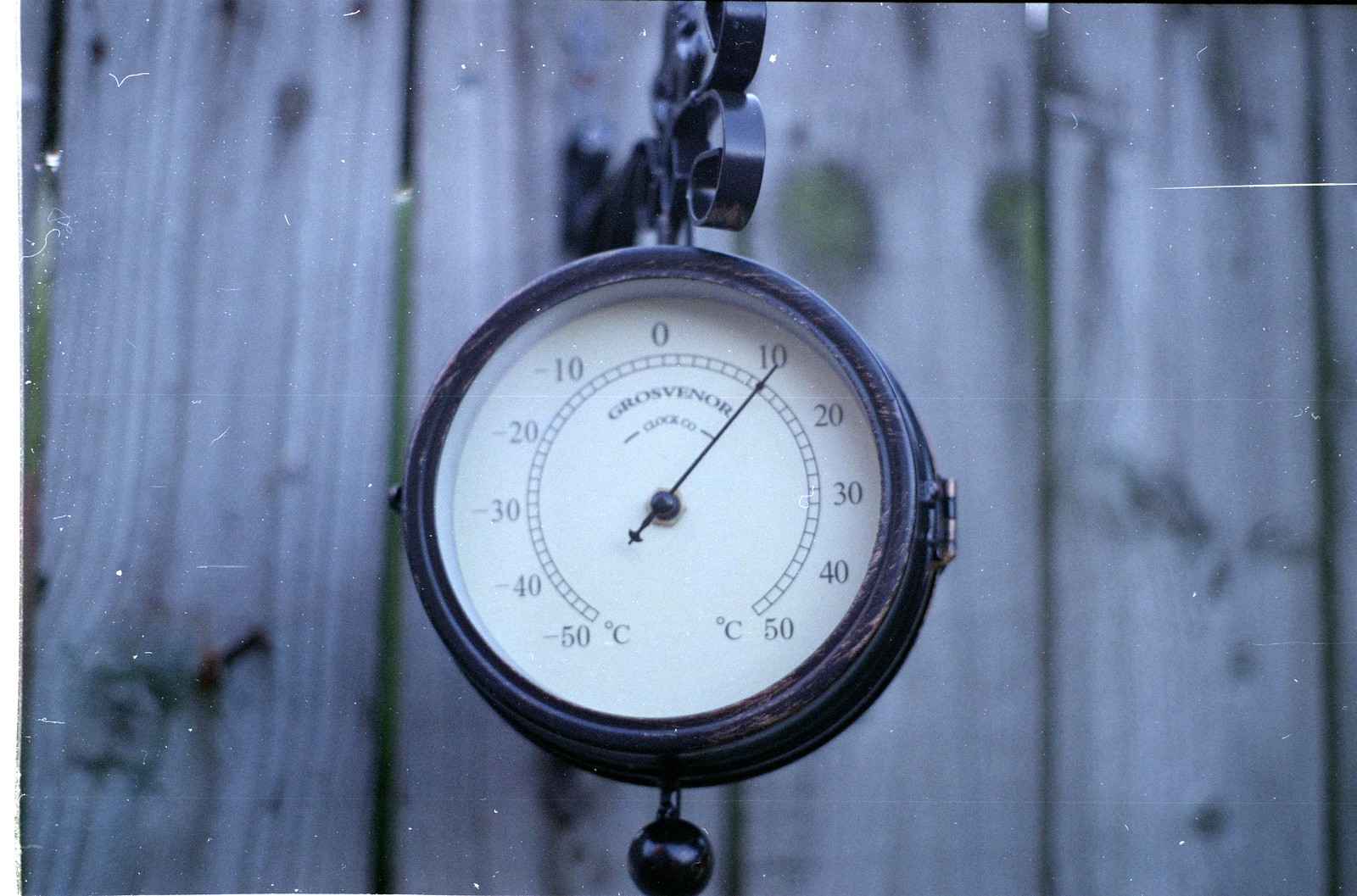In this photograph, an outdoor thermometer is prominently displayed, hanging from an ornate black metal bracket attached to a wooden fence. The fence consists of four vertical, gray-colored posts marked with natural wood knots, enhancing its rustic charm. The metal bracket features an elegant design with loops and curves, which securely holds the thermometer in place.

The thermometer itself is circular, with a bronze and black frame. Its face resembles that of an antique clock, emblazoned with the name "Grosvenor Clock Company." The dial inside features a clean white background, marked with temperature indicators ranging from -50 to 50 degrees Celsius in increments of 10. A single, black needle on the gauge points to 10 degrees, suggesting a chilly atmosphere.

Adding to the photograph’s character, the image comes with a distressed look, showcasing white scratch marks and other weathered effects that appear to be imposed on the image rather than on the actual objects within the scene, lending it a nostalgic and vintage feel.